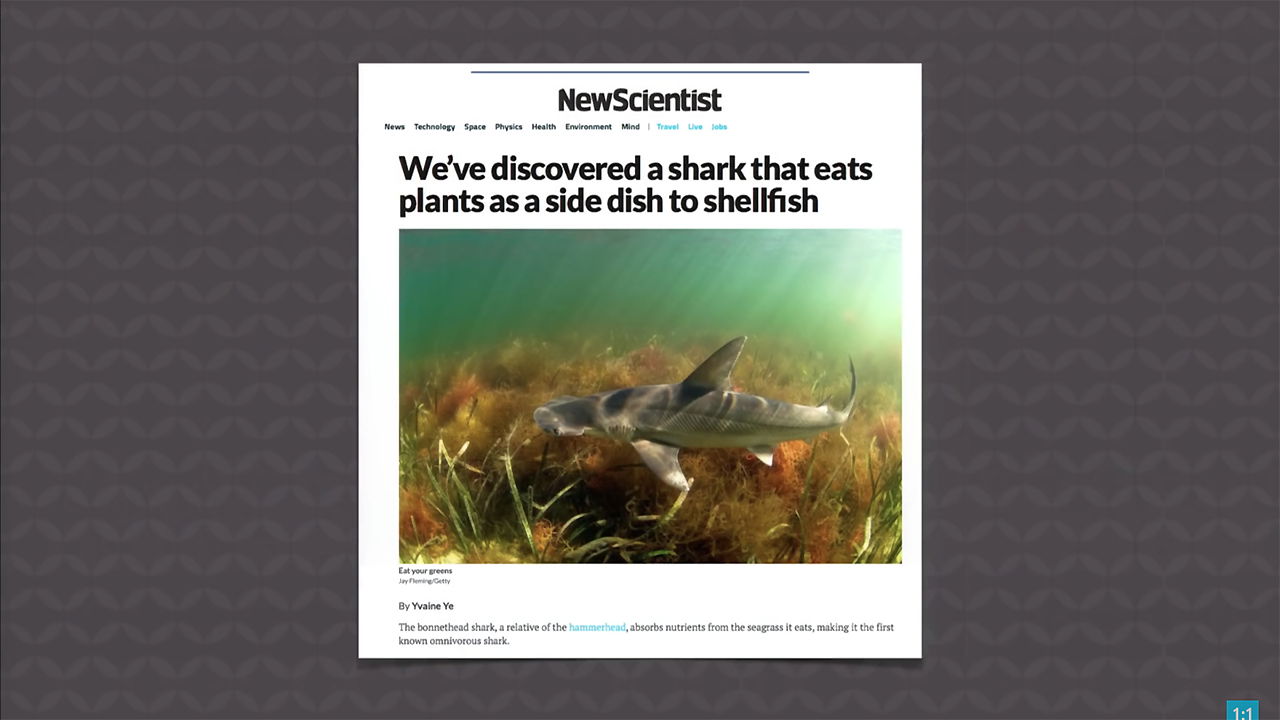The image features a gray background adorned with various light gray lines and shapes. At the center sits a white square, approximately five inches wide and six inches high. At the top of the white square, in black text, it reads "New Scientist." Below this, also in black text, the caption states: "We've discovered a shark that eats plants as a side dish to shellfish."

The main image shows an underwater scene with a greenish hue, illuminated by sunlight streaming down particularly on the right side. The underwater landscape is dotted with low-lying plants in shades of brown and orange, with a few green stems scattered throughout. A small shark with a distinctive triangular gray fin is depicted swimming close to these aquatic plants.

Beneath the image, in small blue text, it reads: "The shark is a relative of the hammerhead, absorbs nutrients from the seagrass it eats, making it the first known shark to do so."